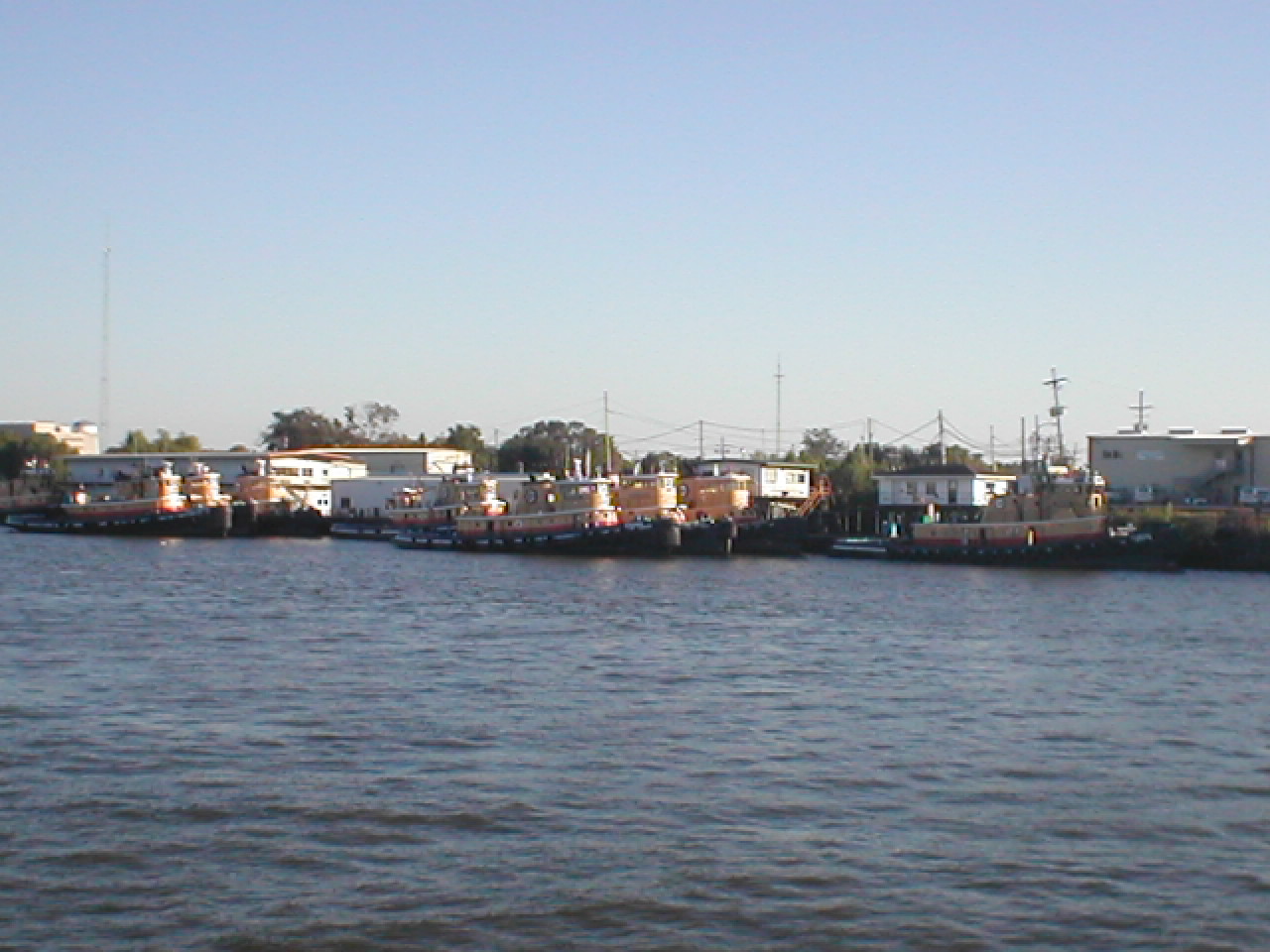This is a detailed outdoor daytime photo of a serene marina. The image captures a calm bay lined with docks and several white buildings. At the forefront, there are multiple tugboats, all uniformly painted with tan wheelhouses and superstructures atop dark brown hulls that extend into the water. The tugboats, six to nine in total, are aligned parallel to one another, with their bows pointing to the right and sterns to the left, indicating they likely belong to the same company. In the background, beyond the tugboats, the scene includes one-story structures, including huts, homes, and industrial buildings on either side of the marina. A two-story industrial building and some trees are visible in the distance, with telephone lines running through the backdrop. The sky is a gradient of blue, lightening towards the horizon, and the calmness of the water beautifully reflects the tranquil atmosphere of the setting.